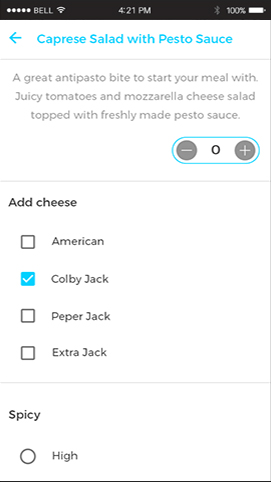The image is a screen grab from a recipe or ordering application, showcasing the details for a "Caprese Salad with Pesto Sauce." At the top of the screen is the dish name, and an arrow points back, suggesting navigation to a previous menu or selection of other salads. Below the title, the description reads: "A great antipasto bite to start your meal with. Juicy tomatoes and mozzarella cheese salad topped with freshly made pesto sauce."

Underneath this description, there's a quantity selector featuring a number (currently zero) flanked by plus and minus icons, allowing users to adjust the quantity of salads to be added to their order. Below the quantity selector, there is an option to add cheese, with four clickable checkboxes: Colby Jack (checked), American, Pepper Jack, and Extra Jack (all unchecked).

Additionally, there is a radio button for selecting a "Spicy High" option, which is currently not selected, indicating that the spicy option has not been chosen for this particular order.